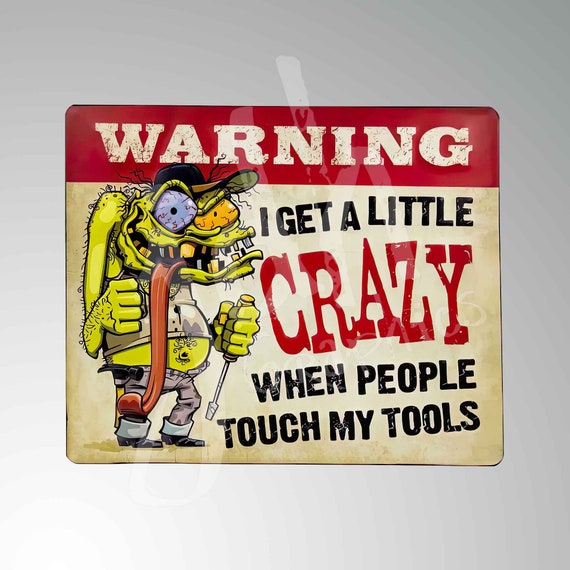The image shows a detailed and vivid sign set against a grayish blue background. At the top of the sign is a red rectangular area featuring the word "WARNING" in bold white capital letters. Beneath this, the majority of the sign is white. 

To the left of the text, there is a menacing cartoon figure depicting a monstrous creature. The creature has green skin and is dressed in a dirty white tank top that exposes its protruding belly, further accentuated by unbuttoned gray pants and black boots. Its face is grotesque, with one bloodshot eye being blue and the other yellow or orange. The creature displays heavily gapped, jagged, yellow and gray teeth, and its mouth is agape, showing a long, curling, red tongue that nearly reaches its feet. It wears a filthy black hat, has scraggly hair scattered across its head and body, including hairy shoulders and arms. The creature holds a screwdriver with a yellow handle and silver flathead tip in its right hand, positioned downward as if ready to stab.

To the right, the sign's text reads, "I get a little crazy when people touch my tools." The word "crazy" is emphasized in large red letters, while the rest of the text is in black. This vivid imagery combined with the bold warning text creates a clear and detailed message suitable for a garage or workshop environment.